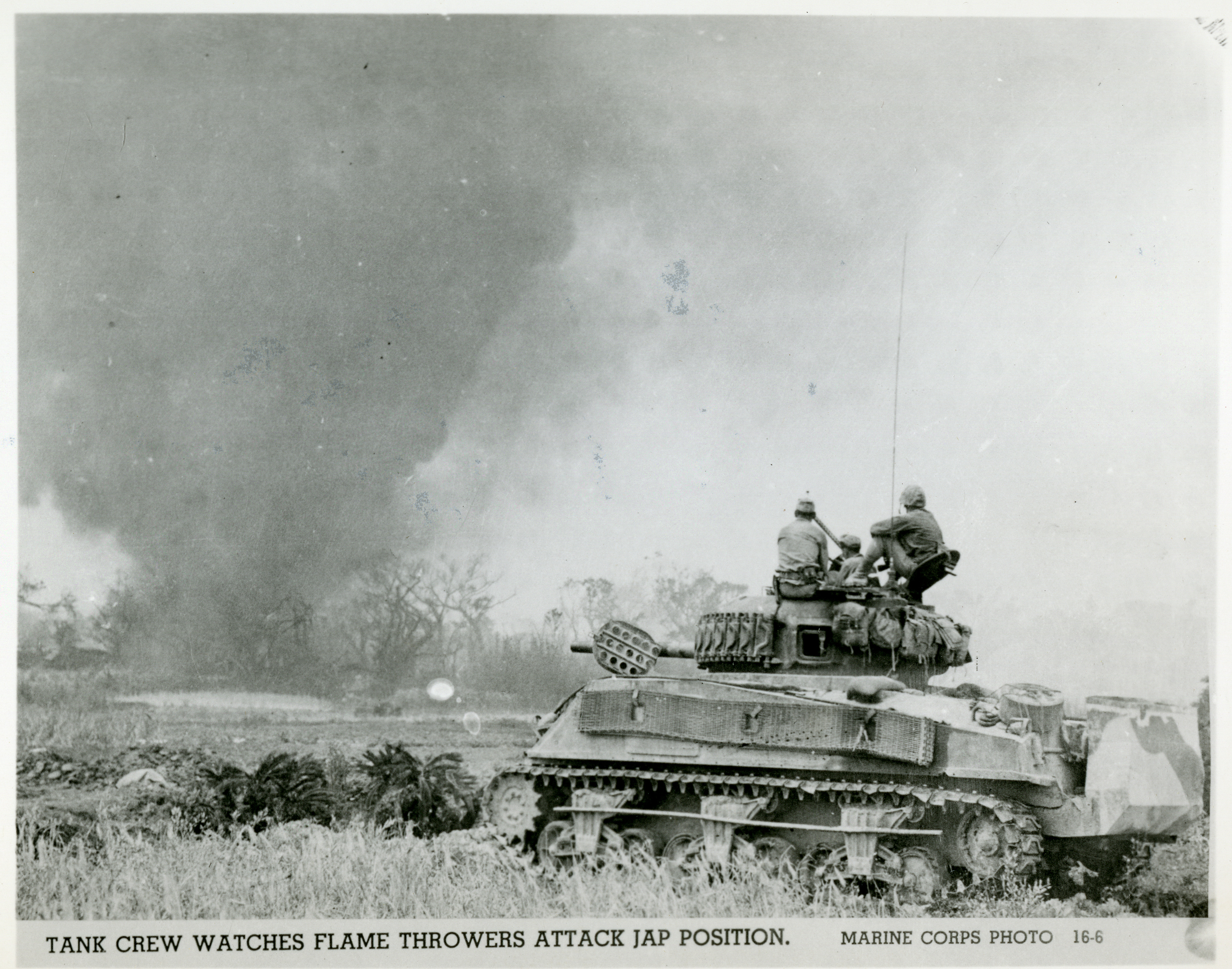This detailed black-and-white photograph, likely taken during World War II, captures a moment on the battlefield. The scene is dominated by a tank positioned prominently in the right-hand corner, with three or four men perched atop it. The label at the bottom of the image reads, "Tank crew watches flamethrowers attack JAP position Marine Corps photo 16-6," which may indicate the date or the photo's sequence in a series. In the background, billowing smoke fills the sky, adding to the sense of chaos and urgency. The ground is sparse, with patches of dry, brown grass and darker, possibly green vegetation scattered around. Bare trees stand in the distance, further emphasizing the stark and war-torn landscape. The overall grayscale of the photo enhances the somber and dramatic atmosphere, with the sky blending into the smoky horizon.